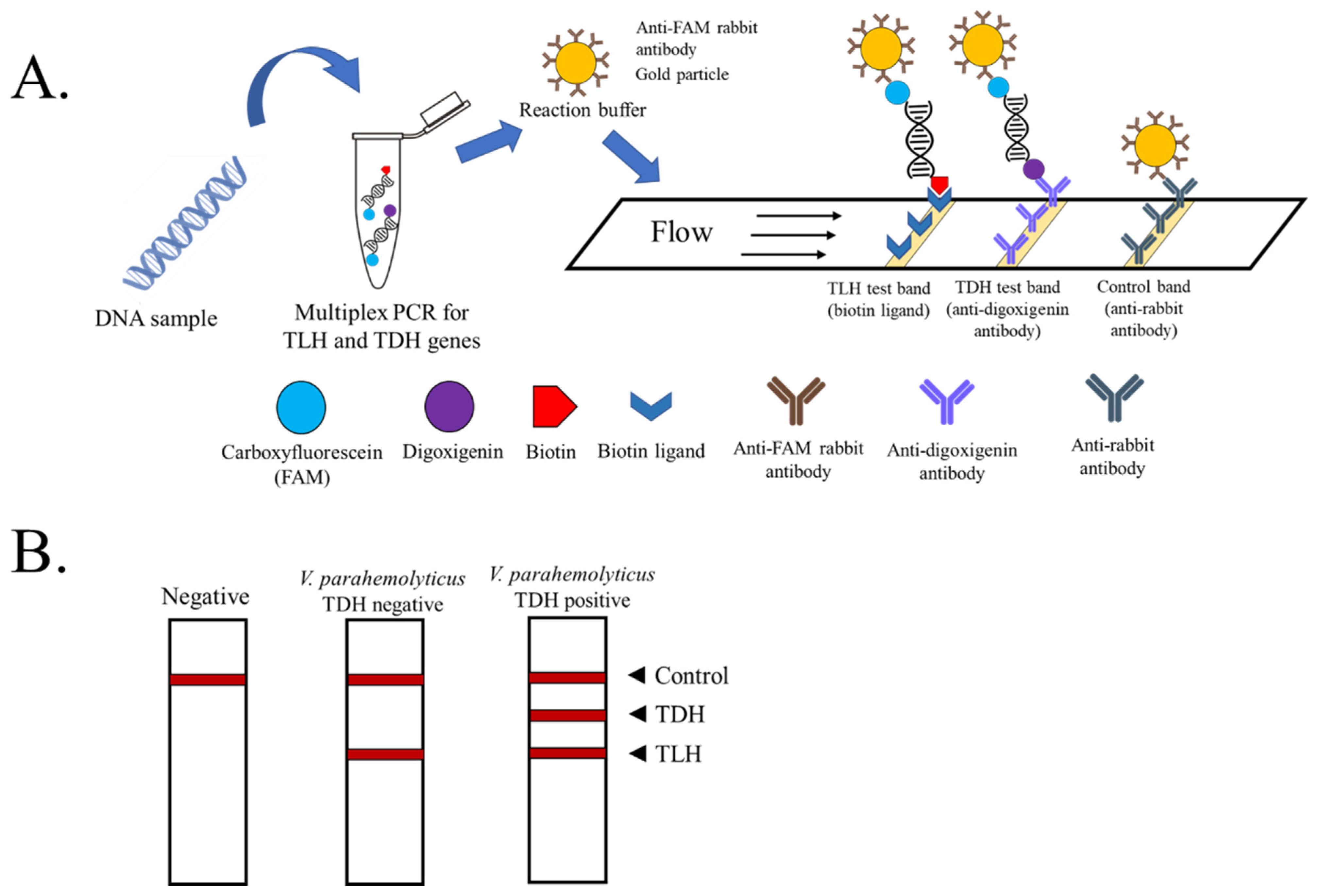The image is a digitally illustrated chart showcasing a scientific explanation involving DNA processing and testing. The chart is divided into two main sections labeled A and B. 

In section A, the image starts with a blue-colored DNA sample being placed into a test tube, labeled "multiplex PCR for TLH and TDH genes." This process is illustrated with a simple double helix icon. The DNA then enters a reaction buffer, depicted as a red sun-like shape with Y-shaped rays extending from it. Following this, the buffered DNA flows into a complex process involving various illustrated cells and scientific components, accented in colors like blue, purple, and red against a primarily white background.

Section B focuses on the results of the testing, showing three test strips. The first strip is marked as "negative" and has a single control line. The second strip labeled "TDH negative" shows two lines: a control line and a TDH line. The third strip, marked "TDH positive," has three lines: a control line, a TDH line, and a TLH line. The results illustrate how the presence of specific lines indicates whether the test is negative, TDH negative, or TDH positive.

Overall, the chart presents a detailed, color-coded process from DNA sampling to result analysis using straightforward illustrations and scientific terminology.